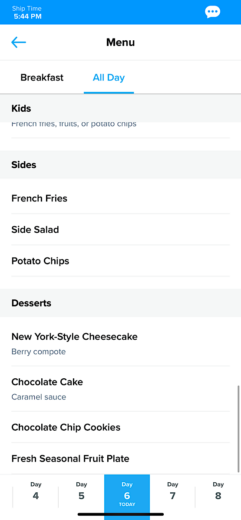This is a detailed screenshot of a mobile app interface.

At the very top, there is a blue bar. On the left side of the bar, it displays in white font, "Ship Time 5:44 PM." On the right side, there is a white chat bubble icon containing three horizontal blue dots.

Below the blue bar, the screen's background is white. At the top of this section, "MENU" is written in black font. To the left of "MENU," there is a blue left-pointing arrow.

Underneath, there is a black horizontal line. Below this line, "Breakfast" is written in black font, followed by "All Day" in blue font. The option "All Day" is selected.

Continuing below, a gray rectangle contains the word "Kids" in black font. Below this, in gray font, it says "French Fries, Fruits, or Potato Chips." 

Next, another gray rectangle with black font reads "Sides," listing "French Fries, Side Salad, and Potato Chips."

Following that, another gray rectangle labeled "Desserts" in black font lists "New York Style Cheesecake" in black font with "Berry Compote" in gray font beneath it.

A horizontal black line separates this section from a new entry below, which reads "Chocolate Cake" in black font, and beneath it, "Caramel Sauce" in gray font.